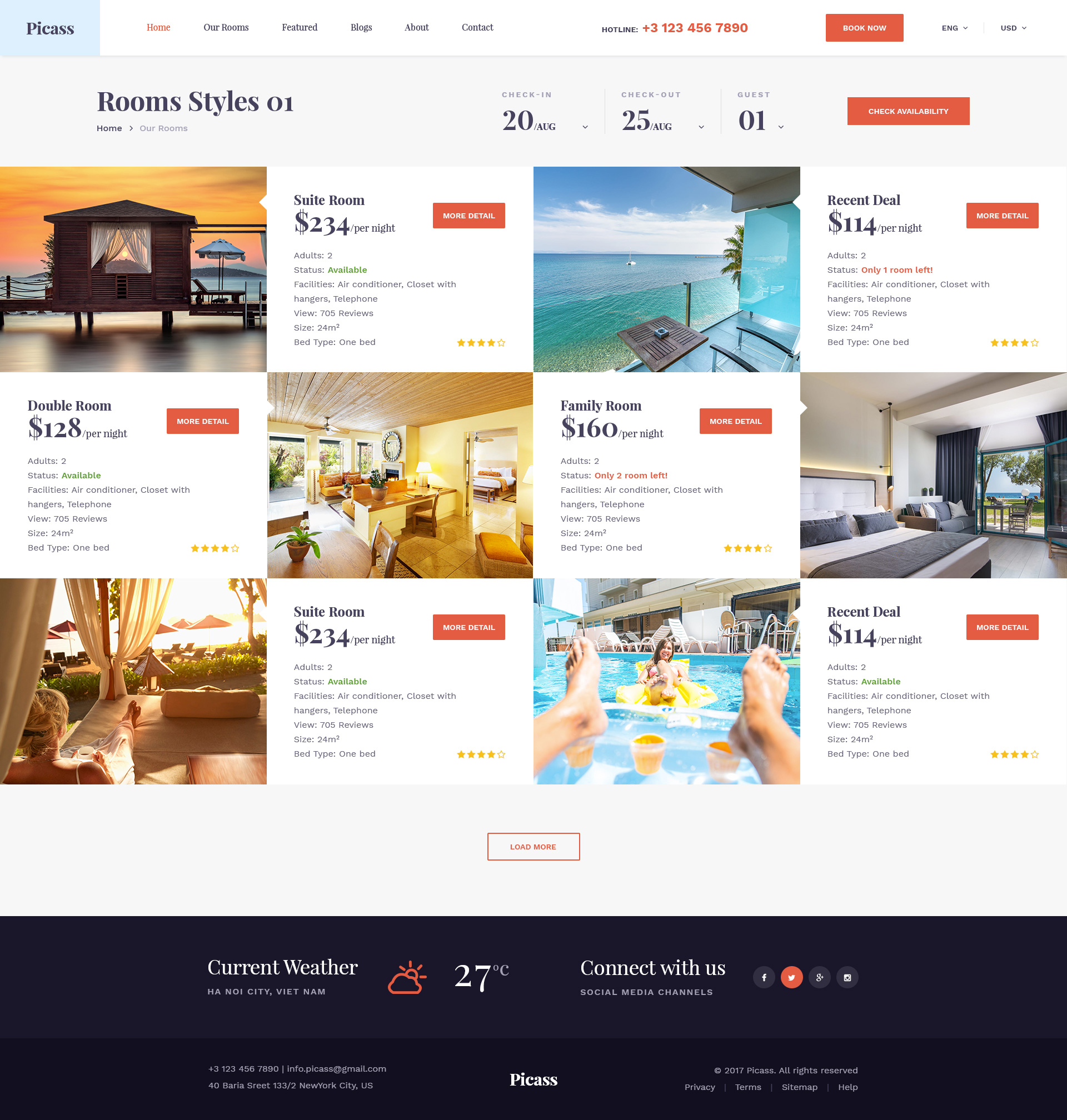Screenshot from Picas Website: Overview of Holiday Locations and Room Types

The image appears to be a detailed screenshot from the Picas website, possibly a property rental or holiday booking site. The site features a comprehensive layout showcasing various holiday locations with numerous rooms available for booking. Here is an in-depth look at its contents:

**Website Overview:**
- **Logo and Navigation:** The upper left-hand corner of the website displays the "Picas" logo within a blue square. A red-highlighted "Home" tab is selected, with additional tabs including "Our Rooms," "Featured Blogs," "About," "Contact." 
- **Booking Options:** A red "Book an Ad" button is prominently displayed, alongside options to customize the website language to English and the currency to US dollars.
- **Search Filters:** Fields to check availability are visible, with inputs for check-in (20th August), check-out (25th August), and the number of guests (1). There is also a "Check Availability" button.

**Room Descriptions:**

1. **Suite Room**: 
   - **Price:** $234 per night
   - **Description:** A hut-like structure on stilts, perched over water with draped curtains, exuding an exotic and serene ambiance.
   - **Details:** 
     - Adult capacity: 2
     - Facilities: Air conditioner, closet with hangers, telephone
     - Room size: 24 square meters
     - Bed type: 1 bed
     - Rating: 4 stars
     - Views: 705 views

2. **Room with Sea View:**
   - **Price:** $114 per night
   - **Description:** Offers a scenic view from the balcony, likely showcasing a slight sea vista.

3. **Double Room:**
   - **Price:** $128 per night
   - **Description:** Features an interior glimpse of what appears to be a kitchen or lounge clad in yellow tones. The bedroom, visible on the right, has large windows or doors with foliage outside.

4. **Family Room:**
   - **Price:** $160 per night
   - **Description:** Furnished with a grey bed adorned with grey and cream cushions and a cover, complemented by grey curtains. The view extends to trees and the sea outside.

5. **Suite Room (Alternate View):**
   - **Price:** $234 per night
   - **Description:** Looking out over umbrellas and deck chairs near the sea, this room projects a luxurious setting. A person with blonde hair is seen relaxing under a canopy, with their legs visible in the lower left-hand corner.

6. **Recent Deal or Suite Room:**
   - **Description:** Middle of the image, showcases a person’s legs resting by the edge of a swimming pool, with a woman on the other side on a floating yellow plastic chair, signifying a relaxed and inviting environment.

The Picas website offers a wide array of aesthetically pleasing and varied accommodation options to potential guests, conveying detailed imagery and room specifications to assist in the selection process.